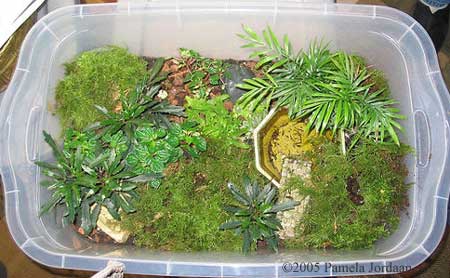This is an overhead photograph taken indoors, showcasing a homemade terrarium housed in a large, rectangular transparent bin, resembling a Rubbermaid-style storage container with two handles on the sides. The terrarium's contents include various green plants, mosses, and potentially some succulents, thinner plants, and different ivies, thriving in the dirt at the bottom. The setting is well-lit and clear, revealing the vibrant greens of the plants inside. Outside the bin, wooden flooring and a shelf or similar structure are visible in the top left corner. The bottom right corner of the image features a copyright mark that reads "Copyright 2005, Pamela Jordan," with "Jordan" notably spelled with two A's.